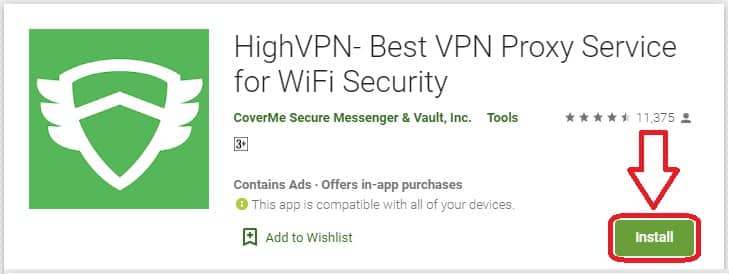**Descriptive Caption:**

This is a screenshot of an application download page for a program called "hi VPN - Best VPN Proxy Service for Wi-Fi Security." The layout is rectangular, featuring a distinctive green and white logo resembling a winged shield within a green square. Below the main title, in smaller green text, it states, "CoverMe Secure Messenger & Vault Inc. Tools." The app boasts an impressive rating of four and a half stars, based on 11,375 user reviews, indicating its popularity and reliability. 

Notably, the application is rated "3+" and includes both ads and offers in-app purchases, as indicated by the accompanying icons. A message with an exclamation mark confirms that "This app is compatible with all of your devices." Users have the option to add the app to their wish list, and there's a prominently featured green "Install" button, highlighted by a red outline and a red downward-pointing arrow, suggesting the next step for interested users.